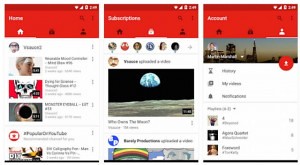The image is a composite of three different screenshots from a video streaming platform, possibly YouTube, organized from left to right: Home, Subscriptions, and Account. Across the top of all three screenshots is a prominent red bar, containing navigational options such as Home, Subscriptions, and Account, along with notification icons.

In the first screenshot depicting the Home screen, there are four video thumbnails showcased, each detailing various content available for viewing. Centrally positioned in this screenshot is a visible username, suggesting the logged-in account.

The second screenshot illustrates the Subscriptions tab. This screen displays a list of channels that the user has subscribed to, alongside previews of two recent videos posted by these subscribed creators. The emphasis suggests an organized feed of new content from preferred channels.

The third screenshot represents the Account page, highlighting the user’s account management options. Here, the history, uploaded videos, notifications, and categorization options for the user's own video posts are visible, arranged in an orderly manner to facilitate easy navigation.

Overall, these three snapshots together provide a comprehensive overview of the platform's key functionalities: browsing general content, following subscribed channels, and managing personal account settings.